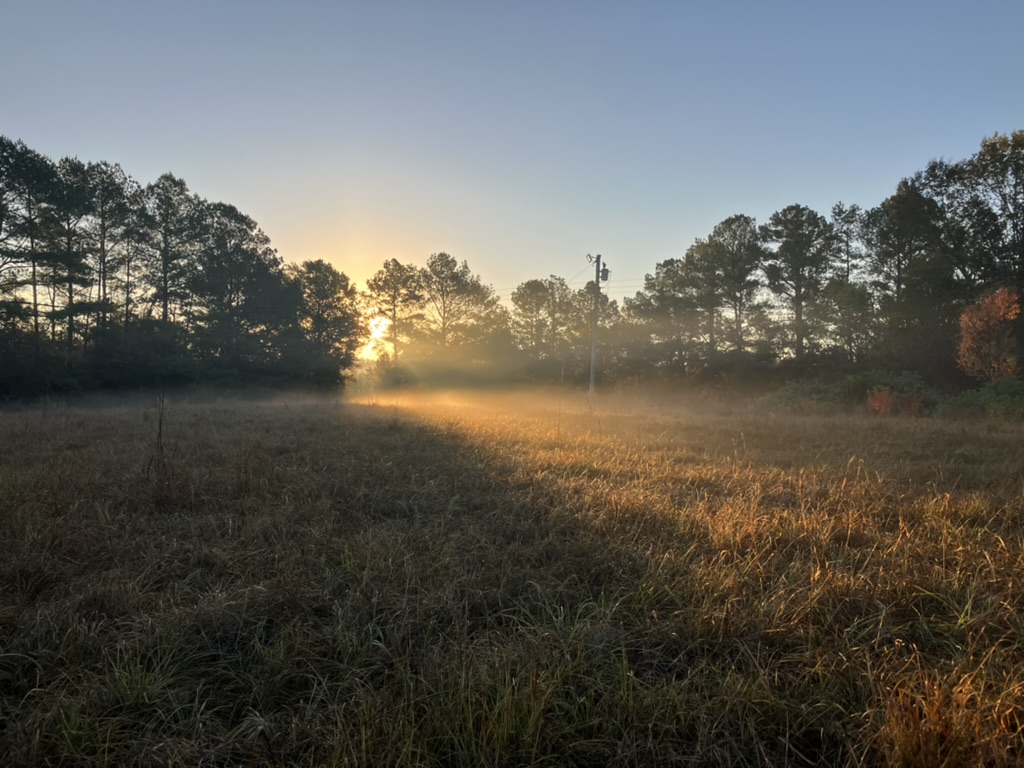This detailed color photograph captures a serene meadow at either sunrise or sunset. Stretching across the foreground is a field of long, somewhat dry grass, painted in hues of brown and green. Where the sunlight touches, the grass transforms into a striking golden color. The center of the image features a yellow sun, radiating light through the trees. The sun’s golden rays illuminate the bottom of the trees, casting a warm glow across the scene. Both sides of the image are lined with trees, mostly covered in green foliage, except for a small tree on the far right, adorned with gold leaves. Near the right of center stands a telephone pole with a transformer, with wires extending to both the left and right. Above this picturesque landscape, the sky exhibits a soft blue hue. The interplay of light and shadow gives the impression of an autumnal setting, capturing the beauty of the moment in vivid detail.